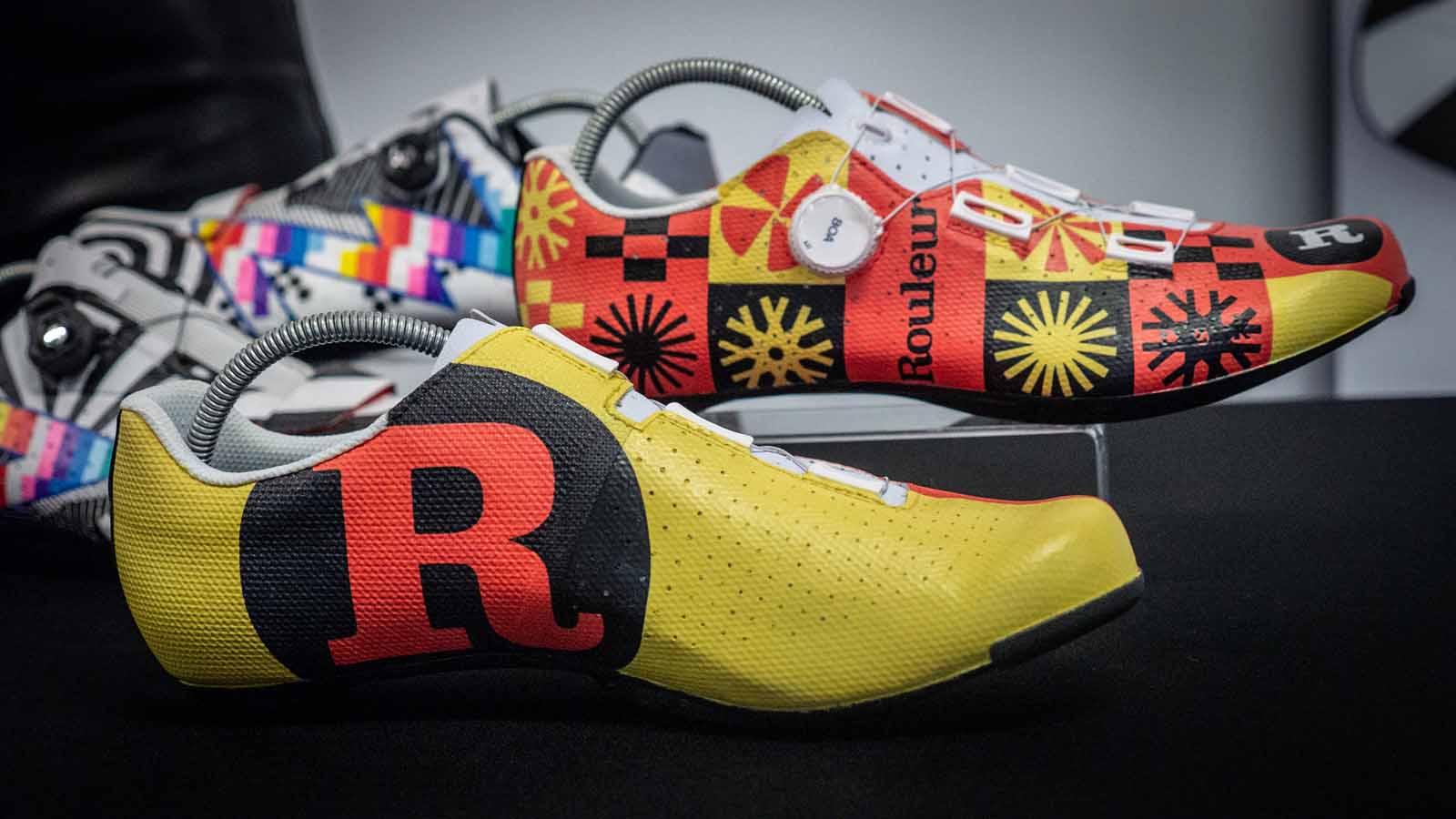In this image, we see two distinctive pairs of shoes placed on a black table against a gray wall. The pair in the foreground is primarily yellow with notable black circles on the side containing red 'R' logos. These shoes lack traditional laces and feature unique designs and minimal soles, possibly indicating specialized athletic or racing footwear. In the background, a white pair of shoes stands elevated on a plastic platform. These shoes exhibit a vibrant array of colors and intricate patterns, including a red, yellow, and black checkered design along with various pinwheel motifs. Text reading "ROLU" is visible on the shoes in the background, adding another layer of detail to their design.